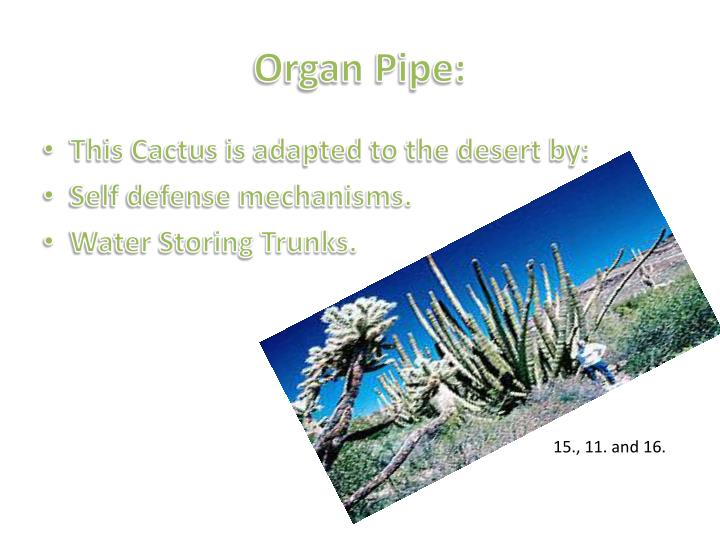On a white background, this illustrated slide showcases an organ pipe cactus. At the top, centered in bold, light green font, it reads "Organ pipe:" followed by three bullet points in a smaller, matching font. The first bullet states, "This cactus is adapted to the desert by:" with a colon. The next bullet point lists "Self-defense mechanisms." The final bullet point mentions "Water storing trunks." A color photograph of a tall, multi-branched cactus, tilted diagonally to the left, features prominently. In the image, the cactus is surrounded by other desert plants under a blue sky, with a person standing beneath it, highlighting the cactus's impressive size. Below this image, in small black font, are the numbers "15, 11, 16."